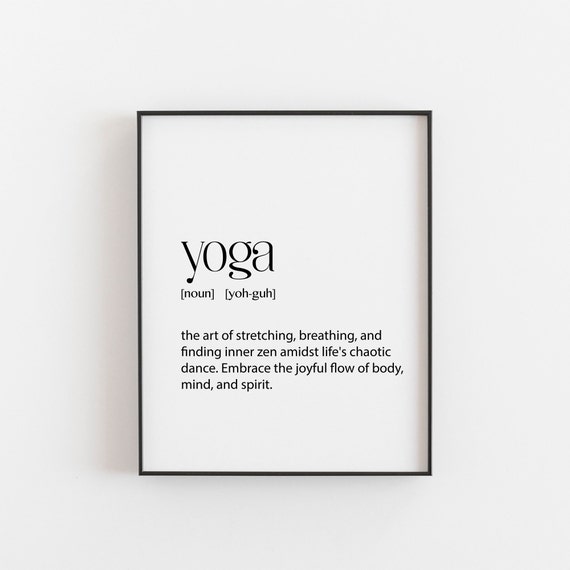The image depicts a minimalist design with a predominantly white background framed by a simple black border. Centered and taking up most of the visual space is a slightly darker grayish-white square. Within this square, the word "yoga" is written in large, dark black lowercase letters, positioned just above the center. Below "yoga," in smaller black font, it states "noun" in parentheses, followed by the phonetic pronunciation "(yoh-guh)". Further down, in black text, is a descriptive paragraph that reads: "The art of stretching, breathing, and finding inner Zen amidst life's chaotic dance. Embrace the joyful flow of body, mind, and spirit." The entire piece uses only variations of black, white, and gray, with no additional graphics or drawings, emphasizing its stark and simplistic aesthetic.